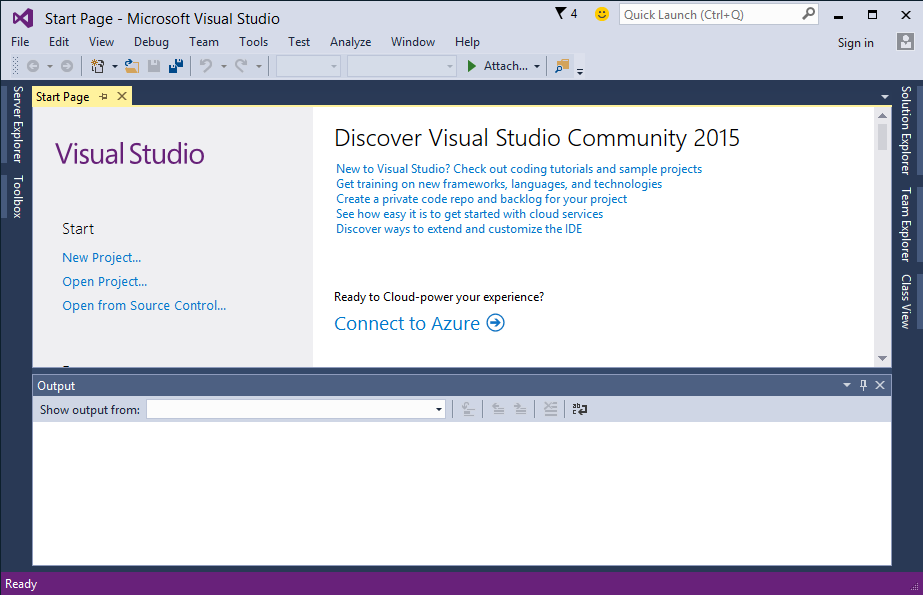The image depicts a computer screen displaying the Start Page of Microsoft Visual Studio Community 2015. The interface features a grey top bar and a black-outlined bottom bar, with the very bottom of the screen shaded maroon. At the top, the title "Start Page - Microsoft Visual Studio" is prominently displayed with a horizontal menu beneath it listing options such as File, Edit, View, Debug, Team, Tools, Test, Analyze, Window, and Help.

Centrally, a section marked "Start Page - Visual Studio" includes options like "Start New Project," "Open Project," and "Open from Source Control." Below this, a large section titled “Discover Visual Studio Community 2015” encourages users to explore coding tutorials, sample projects, new frameworks, languages, technologies, and cloud services. It also highlights how to create a private code repository and backlog for projects, extend and customize the IDE, and connect to Azure for cloud services. A blue arrow within a circle points to the right, drawing attention to the "Ready to Cloud Power Your Experience, Connect to Azure" prompt.

At the bottom part of the interface, under the "Visual Studio" label, there's an "Output" section with a dropdown menu labeled "Show Output From," allowing users to choose specific outputs. The interface features a white area for outputs, and a status message "Ready" appears in the lower-left corner, also in white.